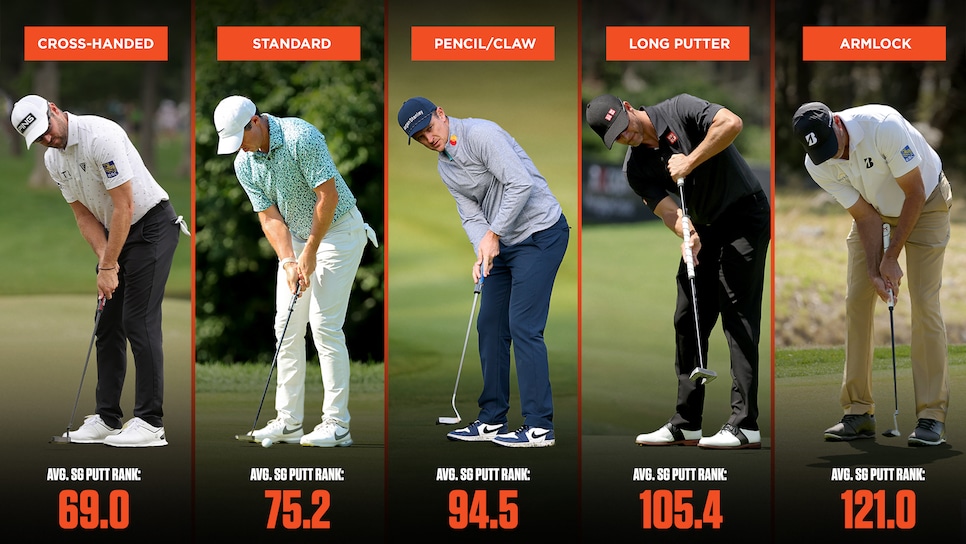This horizontal, rectangular image features five distinct panels, each depicting a different golfing grip style. From left to right, the styles shown are cross-handed, standard, pencil claw, long putter, and armlock. Each panel includes a male golfer demonstrating the corresponding grip on a golf club. 

In the first panel titled "cross-handed," a man dressed in a white jersey, white hat, black trousers, and white shoes is bent over in a putting stance. His putt rank is identified as an average SG of 69.0. The second panel, "standard," displays a golfer with an average SG putt rank of 65.2. In the third panel, "pencil claw," the technique is illustrated by another golfer with an average SG putt rank of 94.5. The fourth panel, "long putter," shows a golfer using this unique grip style with an average SG putt rank of 105.4. Finally, the last panel, "armlock," presents a golfer using the armlock method, marked by an average SG putt rank of 121.0. Each frame offers a visual comparison of the different putting techniques and their corresponding performance metrics.